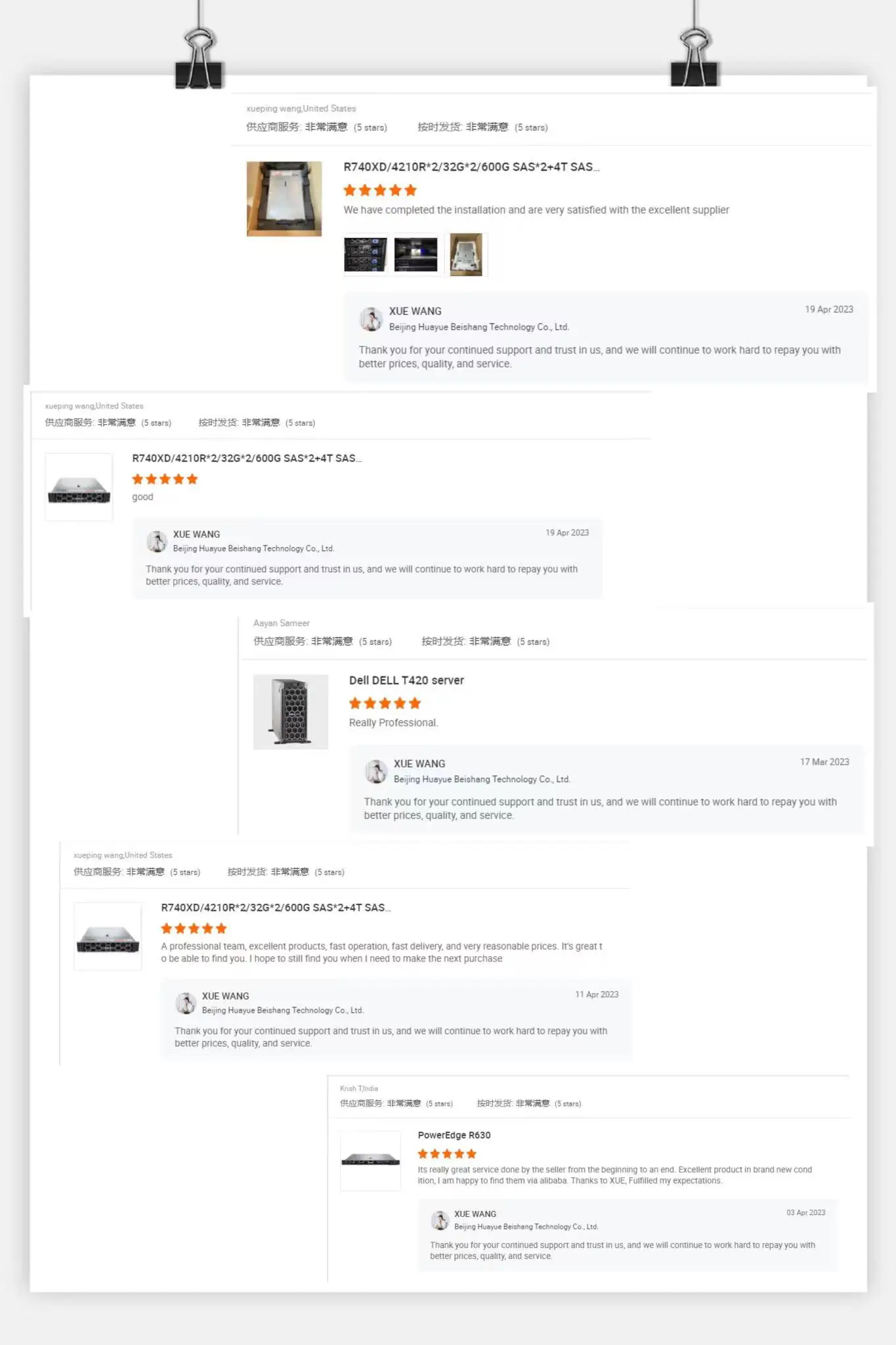Here is a cleaned-up and detailed caption for the image described:

---

The image is a screenshot of multiple five-star reviews on an e-commerce platform dated from March to April 2023. The reviews highlight various customers' satisfaction with high-quality products and services provided by Shu Wang from Beijing Hualaputian Technology Company.

1. Review from Shu Wang, Beijing Hualaputian Technology Company, dated April 19, 2023:
   - Content: The customer expresses complete satisfaction with the installation of their purchase, praising the excellent service and support. They acknowledge the continuous efforts of the supplier to offer better prices, quality, and service.

2. Review from Ayaan Sameer, dated March 17, 2023, for a Dell T420 server:
   - Rating: Five stars
   - Content: The reviewer commends the professional handling of their purchase by Shu Wang, echoing appreciation for the quality and support.

3. Review from Shu Pang Wang, United States, with no specific date:
   - Rating: Five stars
   - Content: The customer highlights the professional team, excellent products, rapid operation, fast delivery, and reasonable prices. They express hope to continue purchasing from the supplier in the future.

4. Review from Tanah Tuta for a PowerEdge R630, dated April 3, 2023:
   - Rating: Five stars
   - Content: The reviewer is very pleased with the service from beginning to end, emphasizing the brand new condition of the product and their satisfaction after finding the supplier via Alibaba.

All reviews conclude with a message from Shu Wang, thanking customers for their continued trust and support, and promising to repay with better prices, quality, and service.